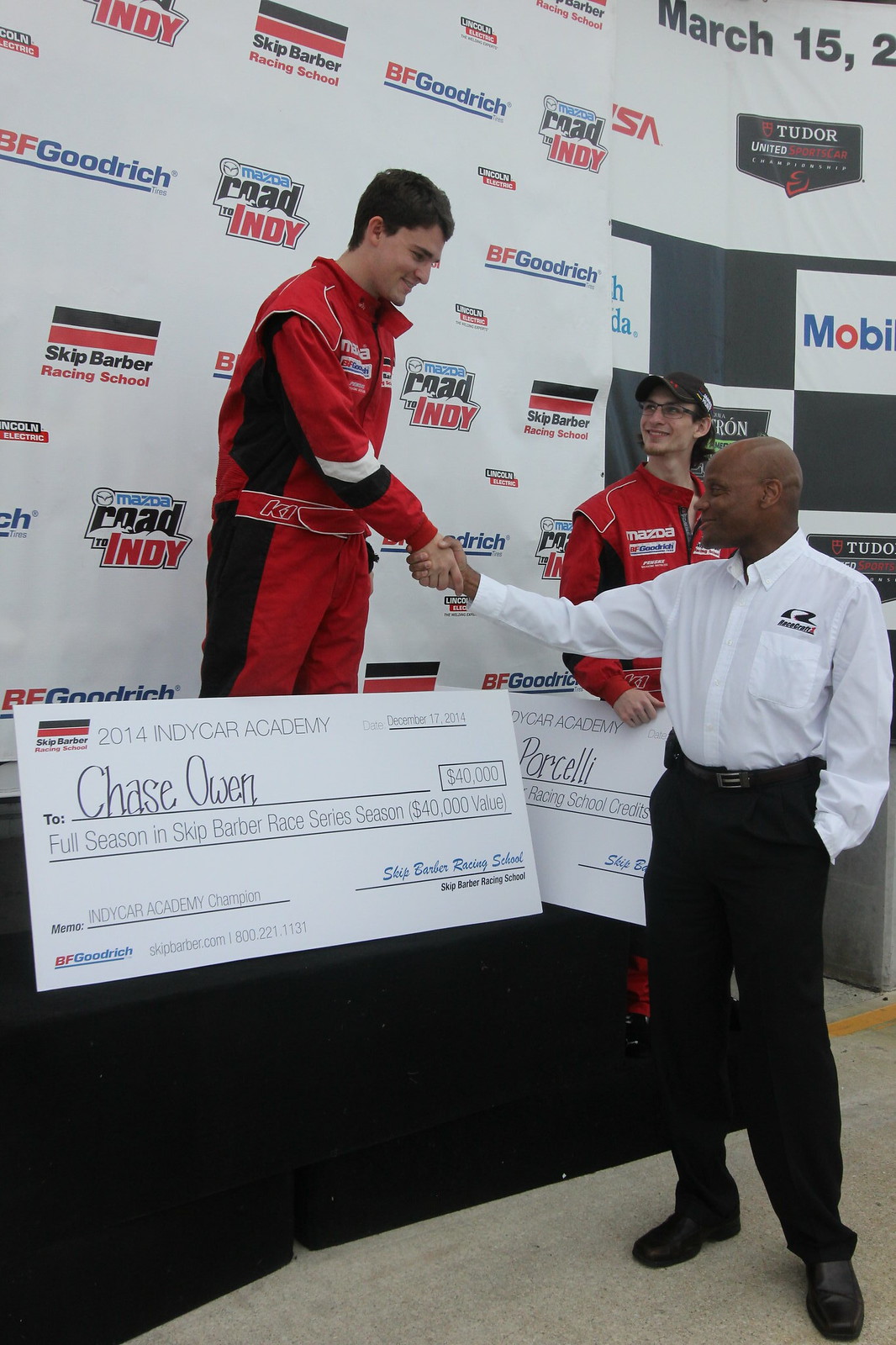In this photo captured at an IndyCar Academy event, a young Caucasian man in his twenties, dressed in a red race car jumpsuit with black accents, sits on a black platform while shaking hands with an African-American gentleman. The man standing below, presenting the handshake, is dressed impeccably in a long-sleeve, white button-up shirt, black pants, and black dress shoes, and has a bald head. The congratulatory moment revolves around a gigantic check positioned near the race car driver’s knees, addressed to Chase Owen for a full season in the Skip Barber Race Series, valued at $40,000. Surrounding the scene are several background signs, including those of BF Goodrich, Road to Indy, and Mobile One, imbuing the photograph with an authentic feel of a celebratory racing event. Additionally, another young Caucasian man, wearing black glasses and a similar race suit, stands to the right of the platform, contributing to the atmosphere of excitement and achievement.